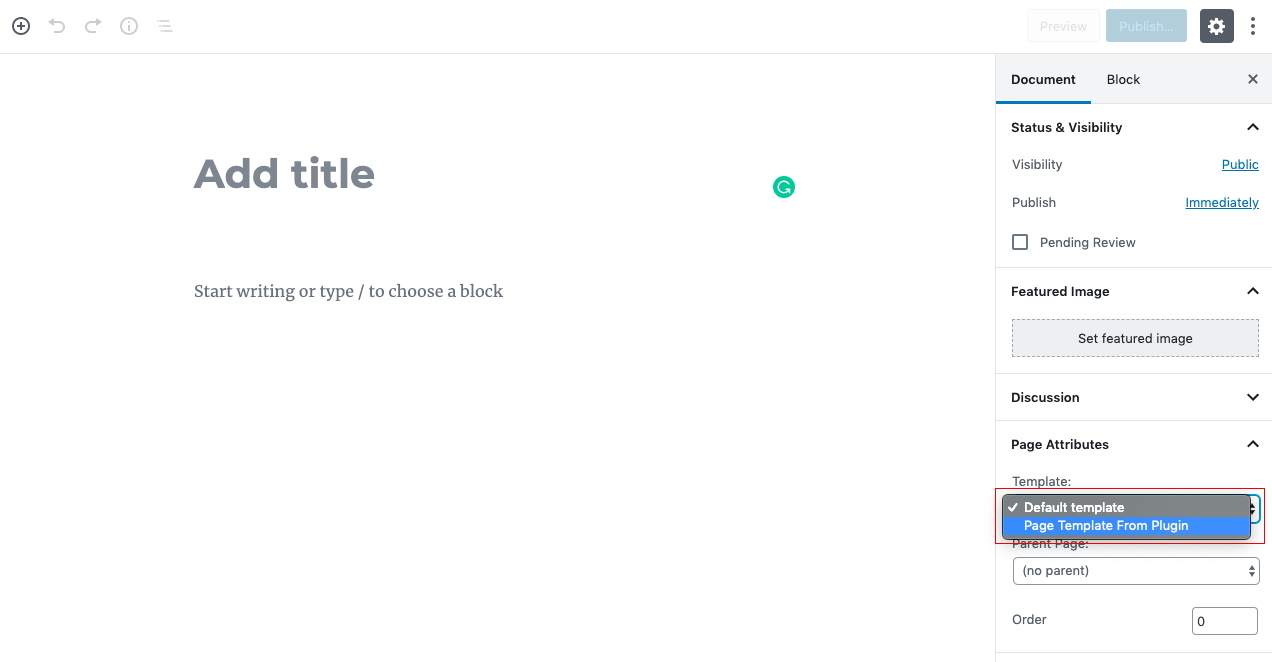The image captures an in-progress presentation slide editor, likely part of an online platform, given the visible interface elements. The slide itself follows a bare-bones template with placeholder text such as "Add title" and "Start writing or type to choose a block." It features a clean, white background and black text. On the right-hand side, a settings pane is visible, indicating options for making the presentation visible to the public or to selected individuals. This pane includes a drop-down menu offering choices between a default template and a page template from a plugin. A box around this section suggests it is currently active or being selected. The pane also shows "Parent page: No parent" and a gear icon in the top-right corner, probably for further settings. Additionally, there is a tab labeled "Block," which likely provides tools for making broader changes to the slide layout or text body.